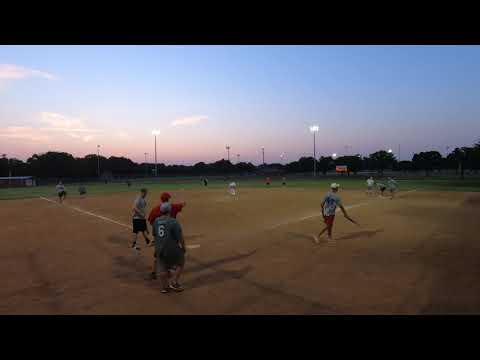This outdoor photograph captures an evening baseball game viewed from behind home plate. The sky, painted with hues of pink and purple, suggests that the sun has just set. Tall, illuminated field lights cast a glow over the scene. The field features a dirt infield and a green outfield, with trees silhouetted against the colorful sky in the distance. The players, mostly men dressed in informal attire of different-colored t-shirts and shorts, are dispersed across the field. Closest to the camera are four players, with others spread out along the baselines and in the outfield. One team appears to be wearing gray, and the other light blue. The umpire, distinguishable by a red hat and red shirt, oversees the game. Amidst the activity, a batter is seen running towards first base, likely having just hit the ball.